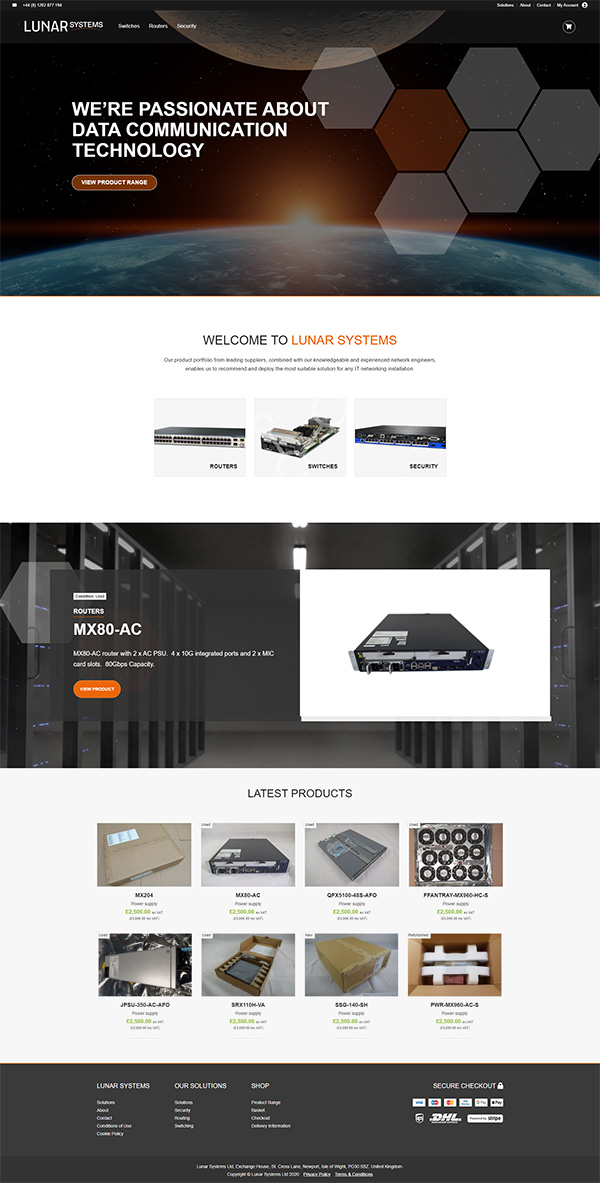### Detailed Caption:

This image captures a screen from a webpage titled "Lunar Systems," prominently reflecting their dedication to data communication technology. At the top of the page, the words "Lunar Systems" appear, emphasizing the brand's focus with a tagline below: "We're passionate about data communication technology." Accompanying this tagline is a clickable button labeled "View Product Range" in a distinctive brownish hue.

In the background, a sliver of the moon is visible at the top, partially cut off, suggesting a celestial theme. Beneath this, a dimly lit Earth occupies the bottom, with sunlight emerging over its middle edge, signifying a new dawn or beginning. The top portion of the screen also features several hexagons, predominantly white, except for a single standout orange hexagon.

Welcoming viewers, the text "Welcome to Lunar Systems" is highlighted, with "Lunar Systems" displayed in orange for emphasis. Below this header are clickable links labeled "Routers," "Switches," and "Security," leading to different sections of the site.

As you scroll down, the page showcases some of Lunar Systems' products under the header "Latest Products." This section displays eight boxed items, each consistently priced at £2,500, with the price mentioned in green within the product descriptions. One highlighted product is the MX204, priced similarly at £2,500.